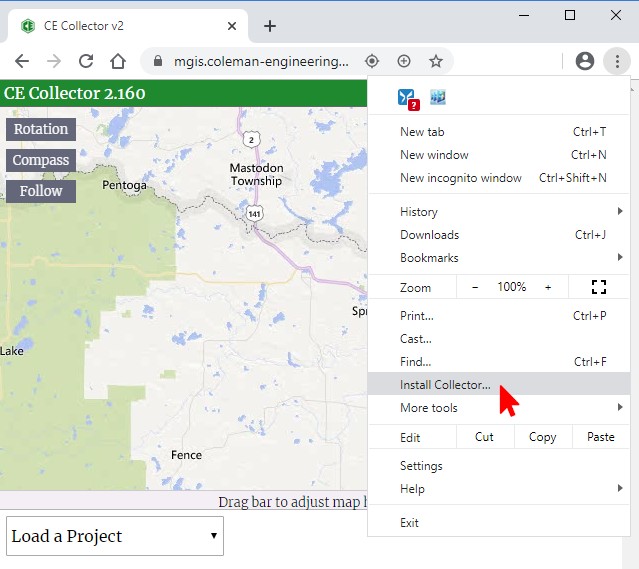Screenshot from a computer displaying the "CE Collector V2" application. The tab in the upper left corner indicates the application name, "CE Collector V2." Below this tab, there is a detailed, zoomed-in map displayed, with a green banner at the top that reads "CE Collector 2.160." 

Overlaying the map are several control buttons including "Rotation," "Compass," and "Follow." Directly beneath the map, there is a drop-down menu labeled "Load a Project." At the bottom center of the map, text reads "Drag bar to adjust map," although this text is partially obscured by an open menu on the right side of the screen.

At the top left of the screen, there are several symbols and a series of textual options, including:
- "New tab (Ctrl+T)"
- "New window (Ctrl+N)"
- "New incognito window (Ctrl+Shift+N)"
- "History"
- "Downloads (Ctrl+J)"
- "Bookmarks"
- "Zoom 100%"
- "Print (Ctrl+V)"
- "Cast"
- "Find (Ctrl+F)"
- "Install collector" (highlighted in a gray box with a red arrow pointing to it)
- "More tools"
- "Edit"
- "Cut"
- "Copy"
- "Paste"
- "Settings"
- "Help"
- "Exit"

This menu provides various navigation and tool options for enhancing user interaction with the application.